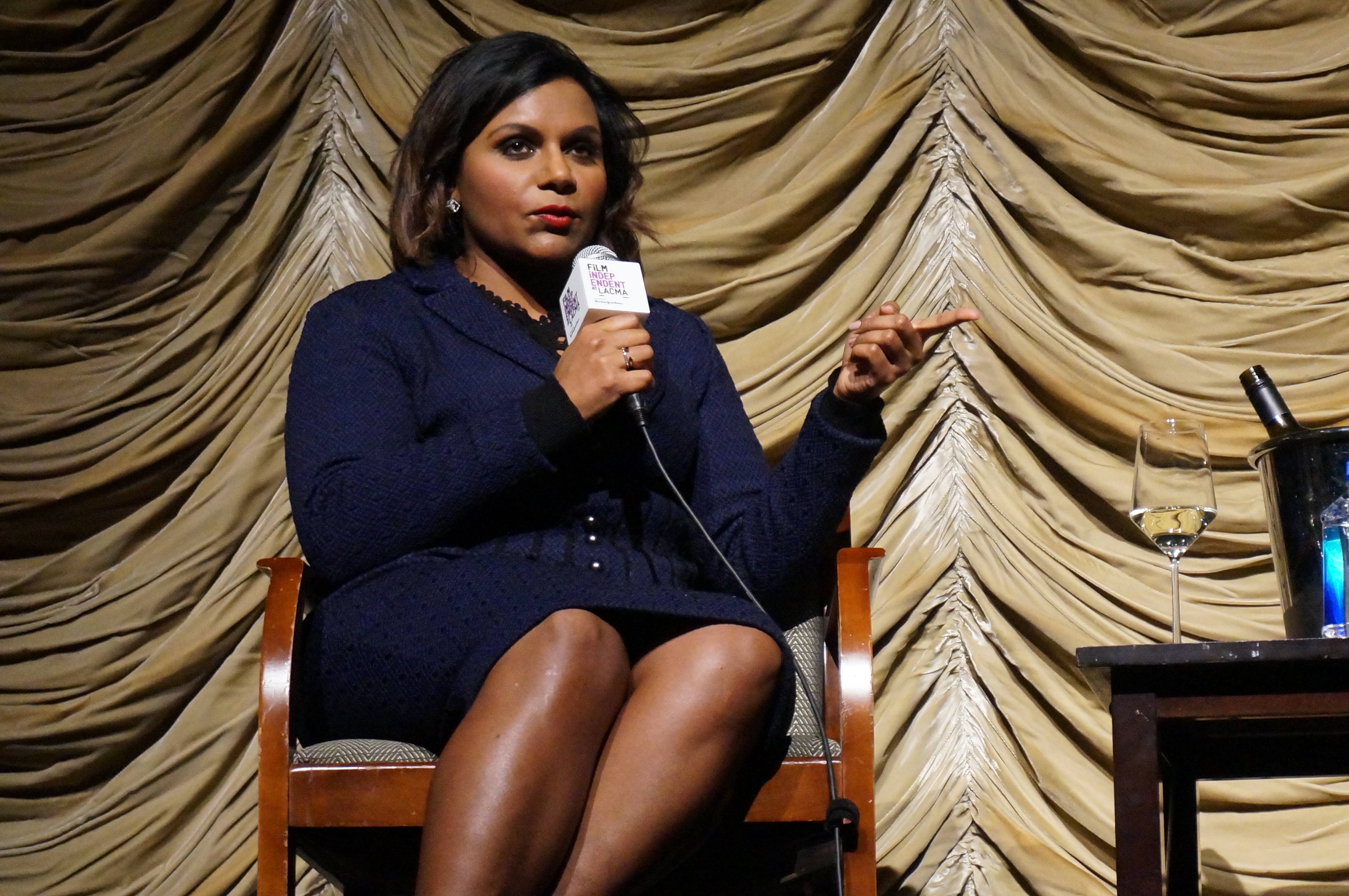A woman is captured on stage during a speaking event, seated in a reddish-brown wooden chair with gray cushions. She is dressed in a dark blue business suit with silver buttons and a matching skirt, complemented by a black top underneath visible at the wrists. The woman is holding a microphone with a distinctive large white box around its handle and is actively gesturing towards the right. A small brown coffee table to her left bears a wine glass filled with clear liquid and a black wine bucket, from which the neck of a wine bottle protrudes. The stage’s backdrop features a tan-colored draped curtain, adding to the formal setting. She also wears rings which add a subtle touch of personal style to her professional outfit.